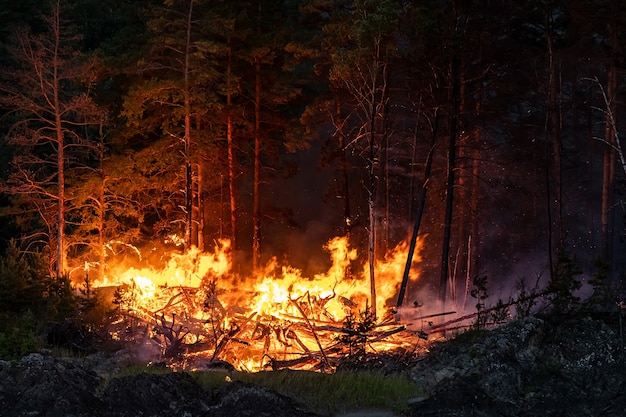This is a detailed photograph capturing the initial stages of a forest fire at night. The image centers on a clearing in the forest, where flames from what appears to be an out-of-control campfire grow in intensity, forming a sizeable blaze equivalent to five to eight campfires merged together. Surrounding this inferno are trees that look mostly deciduous, with a few coniferous ones, possibly pines, in the mix. Several trees on the edges of the clearing are already charred and show signs of burning. The fire's light starkly illuminates some of these trees, half of which are leafless, suggesting they might either be dead or it could be wintertime. The ground in the foreground features green grass, rocks, weeds, and brush that are beginning to catch fire. There is also visible blackened, charred remains of burnt trees scattered about. Smoke mixed with ash or dust billows out to the right, adding a gray haze to the dark night sky. The overall mood is ominously accentuated by the dark backdrop, with white specks—possibly ash or even snow—drifting through the night.